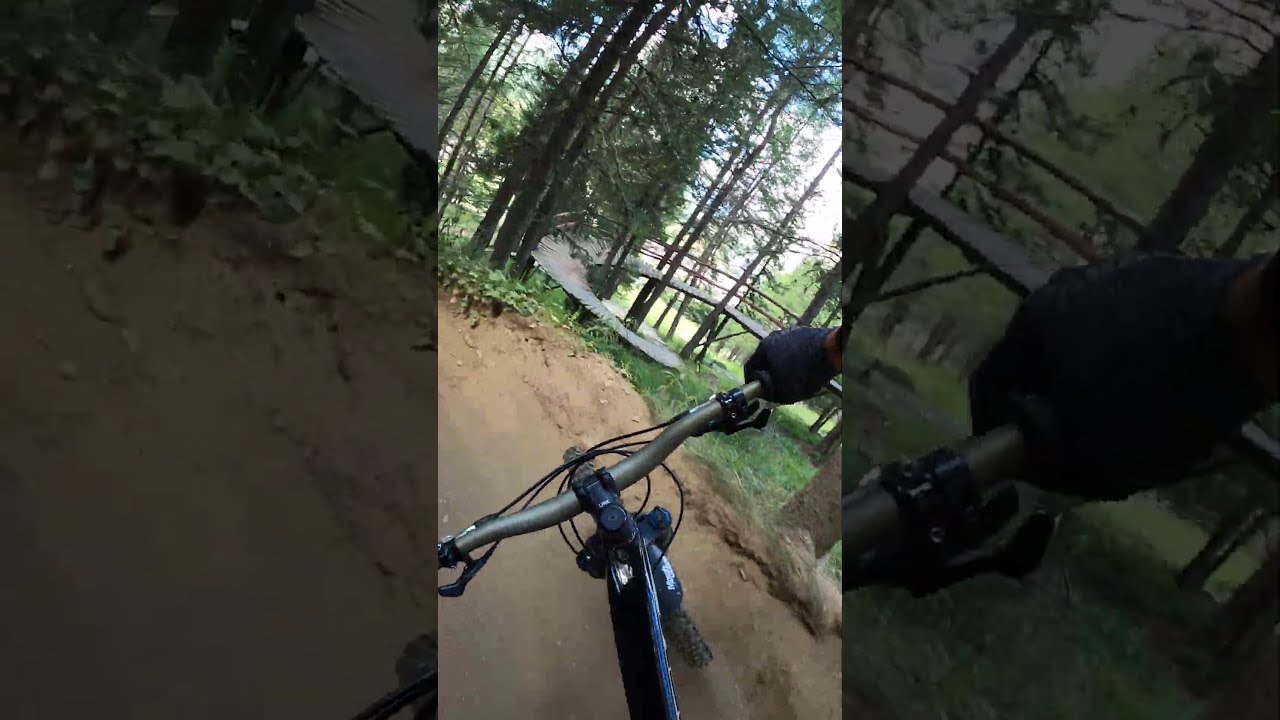The image captures a first-person perspective of someone riding a mountain bike along a compacted, light brown dirt road. The center of the image prominently features the bike's black frame with silver handlebars, both gripped by hands clad in black gloves. The outskirts of the road are lined with dense, dark green vegetation and towering trees with dark brown trunks and foliage. In the distance, a wooden ramp with brown railings curves clockwise to the right and connects to the trees. The photo exhibits a unique composition, with the central area brightly illuminated, while the left and right sides are darker and somewhat out of focus. The right side emphasizes a zoomed-in view of the gloved hand gripping the handlebar, and the left side showcases a close-up of the ground foliage and part of the ramp.